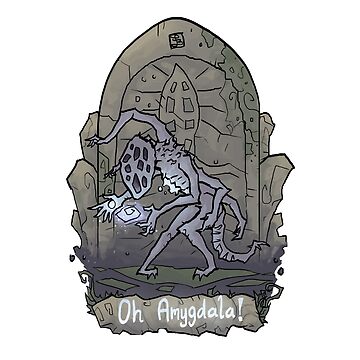The image is a detailed cartoon drawing of a tombstone, set against a stark white background, giving it a minimalist yet eerie appearance. The tombstone, gray and rock-like, has a jagged, curved top and is riddled with cracks, with a noticeable crumbling section at the top right corner. Intricately carved into the stone is a design that resembles either a rocket ship or an alien spaceship, embellished with beams or additional cracks emanating from its sides.

Standing on a green and black surface in front of the tombstone is a monstrous creature, depicted in a lighter gray shade. This alien-like creature has an array of distinct features: it possesses six arms, two legs, and a tail. One of its arms emerges from its back with a sharp hand, while another holds a device featuring a white dot in its center. The monster’s head is characterized by a multitude of black tile-like pieces, giving it a sinister appearance. Between its hands, the creature holds a glowing, diamond-shaped swirl object.

Beneath this detailed scene, the words "O Amygdala!" are inscribed in bold white letters, serving as a prominent exclamation. The haunting composition is completed with a square symbol adorned with an abstract design situated at the top of the tombstone. Overall, the drawing combines elements of sci-fi and horror, creating a uniquely captivating image.